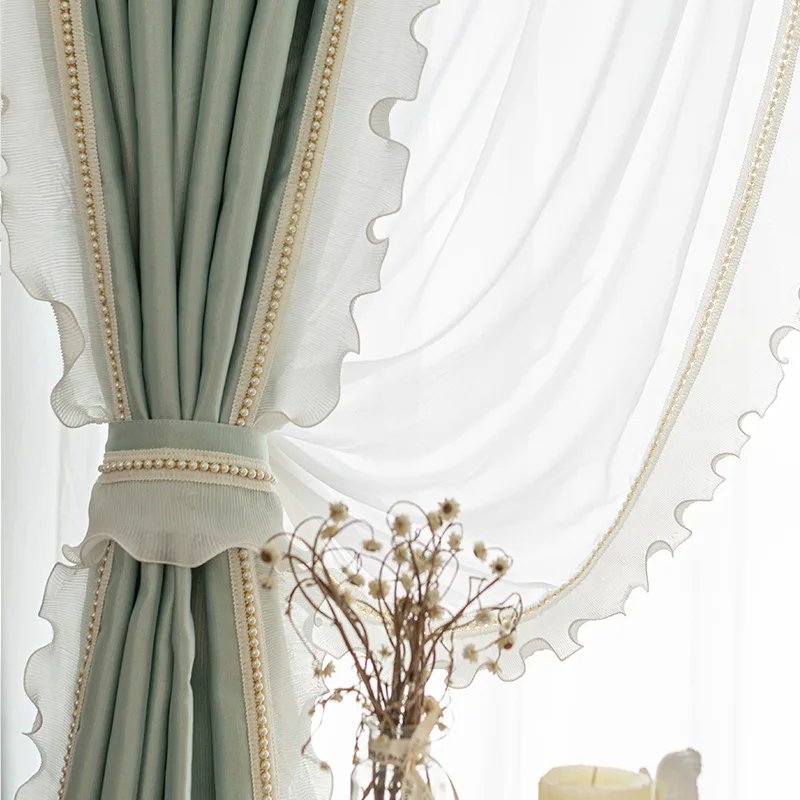This photograph captures an elegantly arranged window featuring a series of ornate and professionally styled curtains. The primary curtain, tied back in an old-fashioned yet sophisticated style, is a thick, heavy lime green fabric with gold-threaded decorative edges. This curtain is held by a matching green tie embellished with an ivory bead pattern, allowing light to filter through a sheer white curtain beneath it. This innermost white curtain, adorned with pearls and lace, partially covers the window to allow natural light, whereas fully unwrapping the green curtain would result in complete darkness. Flanking the composition is another decorative white curtain with a ruffled edge, adding to the layered and ornate aesthetic. Situated in front of these meticulously arranged curtains is a small bouquet of dried flowers, possibly cottonwood branches, complemented by the top of a candle, adding a touch of rustic charm to the overall scene.